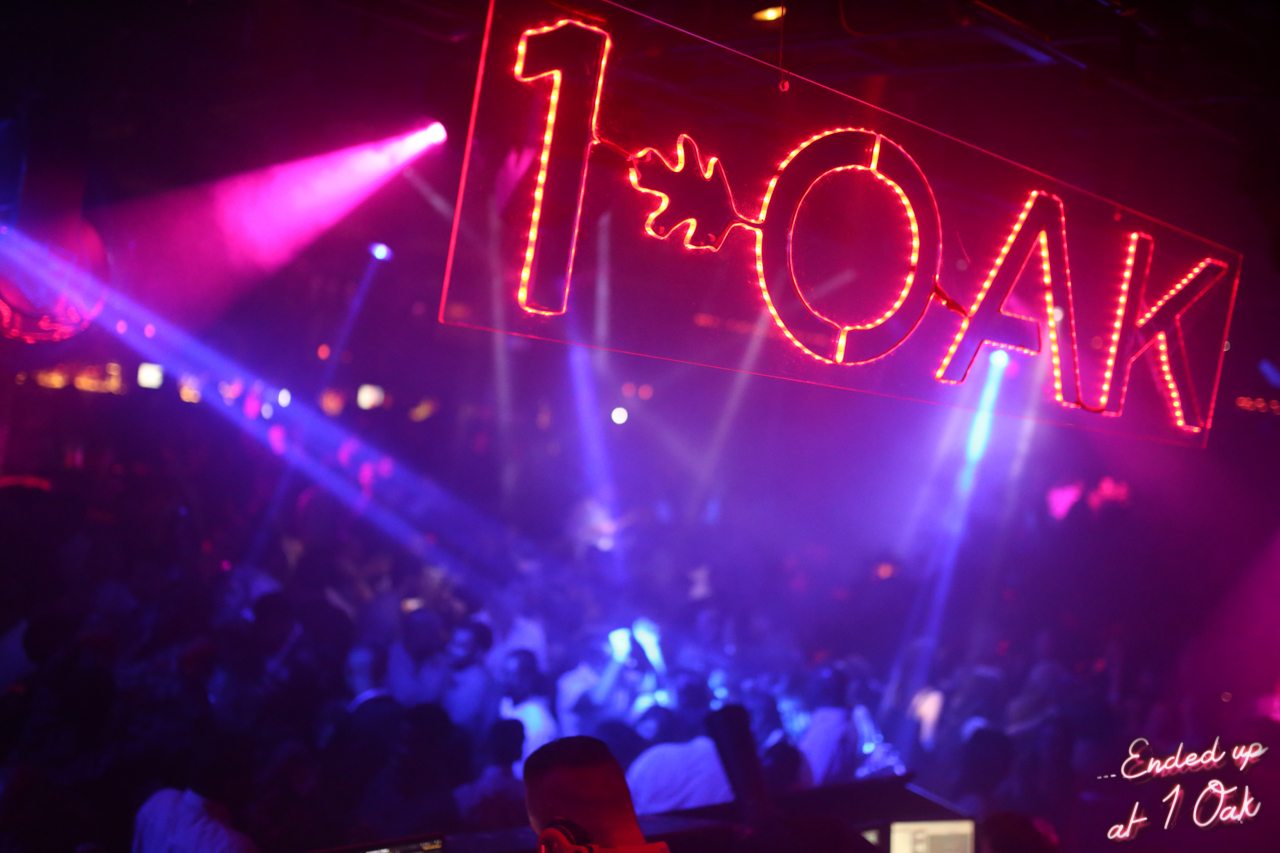The image captures a vibrant nightclub scene, focused on a large, eye-catching sign that reads "1 Oak." The sign, possibly made of glass, is rectangular in shape, about 3 to 4 feet long and 1 foot high, and features a leaf design between the words "1" and "Oak." The text and design are illuminated with yellow LED lights. It hangs above the DJ booth, where only the DJ's head is visible, silhouetted against the backdrop of colorful spotlights in shades of red, blue, pink, and green. The dance floor beneath the sign is bustling with numerous party-goers dancing amid the roving lights. In the bottom right corner of the image, the caption "Ended up at 1 Oak" is written in a glowing, shaded font, angled slightly upwards to the right, adding a final touch to the lively scene.